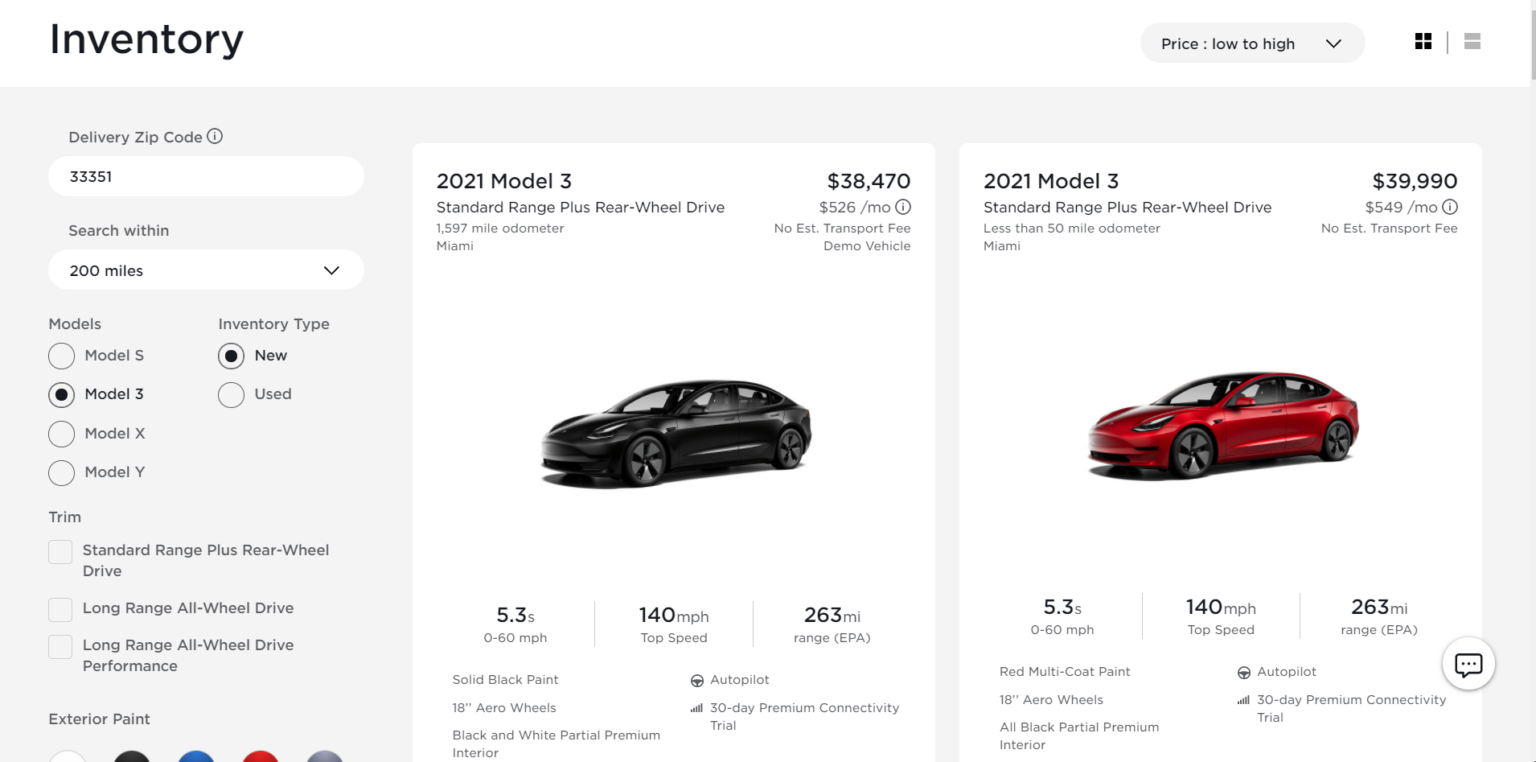This image showcases a website focused on car sales, specifically featuring a vehicle inventory filtering page. At the top left corner of the image, the word "Inventory" is prominently displayed, indicating the section of the website being viewed. On the top right, a sorting option labeled "Price: Low to High" is visible, accompanied by a down arrow for further sorting options.

On the right side of the image, there are two clickable square boxes with white backgrounds, each representing a different car for sale. The left box displays a black 2021 Model 3. At the top of this box, "2021 Model 3" is listed along with its corresponding price, "$38,470," and a financing option of "$526/month." A photo of the black car is shown, positioned diagonally toward the bottom left of the frame. Beneath the car, three key performance stats are highlighted: "5.3 seconds" (likely 0-60 mph acceleration), "140 miles per hour" (top speed), and "263 mile range" (maximum driving range on a full charge).

Adjacent to it, the right box features a red 2021 Model 3 with similar layout and information. The vehicle is also positioned diagonally, mirroring the black car's orientation. The price listed for this red car is "$39,990," with a monthly payment option of "$459/month." Despite the difference in price, the red car shares the identical performance stats: "5.3 seconds" acceleration, a top speed of "140 miles per hour," and a "263 mile range."

These comparative listings offer potential buyers a detailed view of different vehicle options, pricing, and performance specifications.